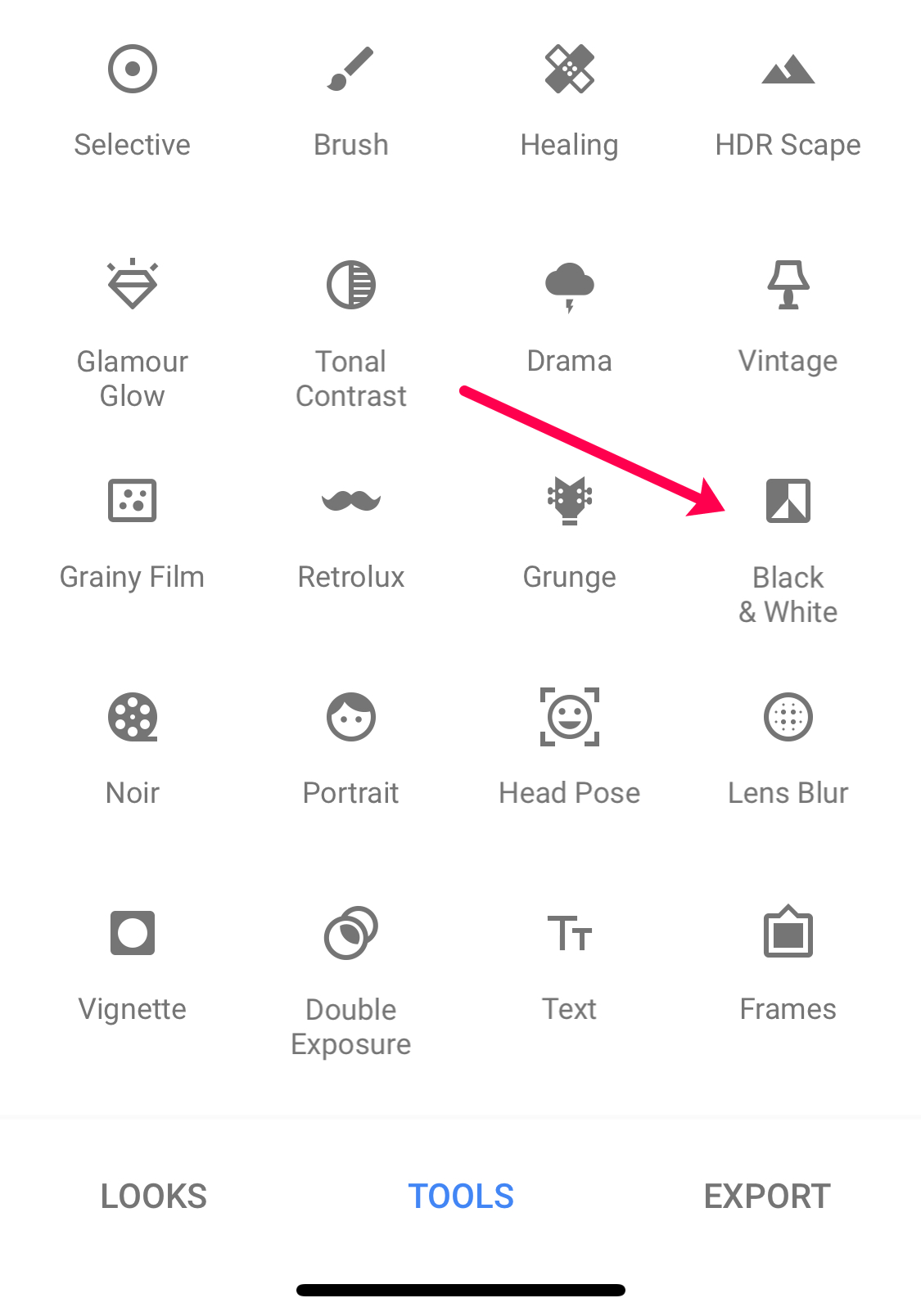In this image, we see a screenshot from a photo editing application. Dominating the bottom section of the picture, there is a black menu bar featuring three options: "Looks," "Tools," and "Exports." The "Looks" and "Exports" options are written in grey ink, whereas "Tools" is highlighted in blue ink, indicating that the "Tools" menu is currently active. 

Beneath this menu, a black underline visually emphasizes that the "Tools" section is selected. The rest of the screenshot is rendered in shades of grey, giving it a monochromatic appearance, which includes both the text and icons delineating various editing functions.

The "Tools" menu displays an array of editing options including "Selective," "Brush," "Healing," "HDR Scape," "Glamour Glow," "Tonal Contrast," "Drama," "Vintage," "Grainy Film," "Retrolux," "Grunge," "Black and White," "Noir," "Portrait," "Head Pose," "Lens Flare," "Vignette," "Double Exposure," "Text," and "Frames." 

An arrow is prominently pointing towards the "Black and White" option in the list, signifying it as the focus or perhaps the next step the user is expected to take.